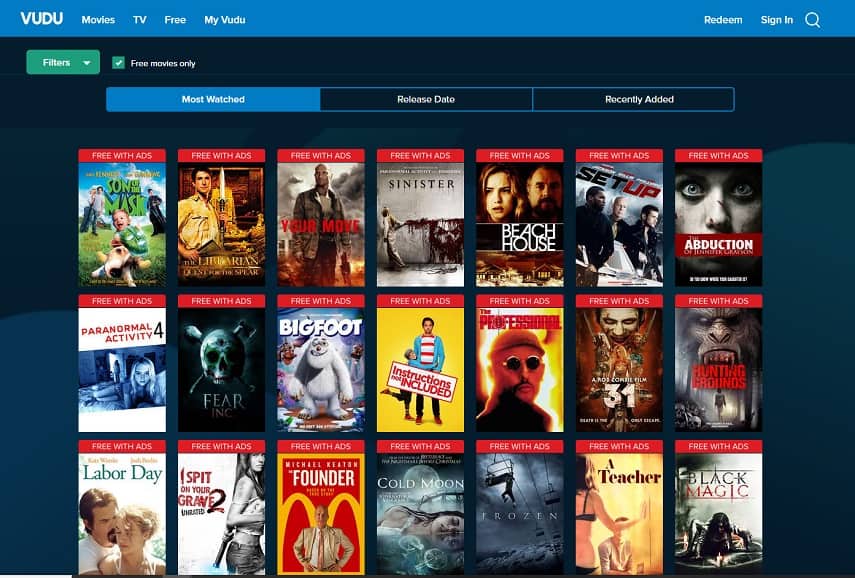This image showcases the main page of the VUDU website. At the top, a light indigo blue border extends across the page. On the left side of this border is the VUDU logo in white. Moving rightward, the menu items read: "Movies," "TV," "Free," and "My VUDU." At the far right of the same border, options to "Redeem" and "Sign In" are displayed, along with a search bar.

Beneath the VUDU logo on the left side of the page, there is a green "Filters" button accompanied by a checkbox labeled "Free Movies Only," which is currently selected. Below these filters, three tabs are visible: "Most Watched," "Release Date," and "Recently Added," allowing users to sort the movie listings accordingly.

The main content of the page features three rows of movies, each row containing seven movie titles. Each title is represented by its cover art or movie poster, neatly organized in a grid format, presenting a clean and organized interface for browsing.